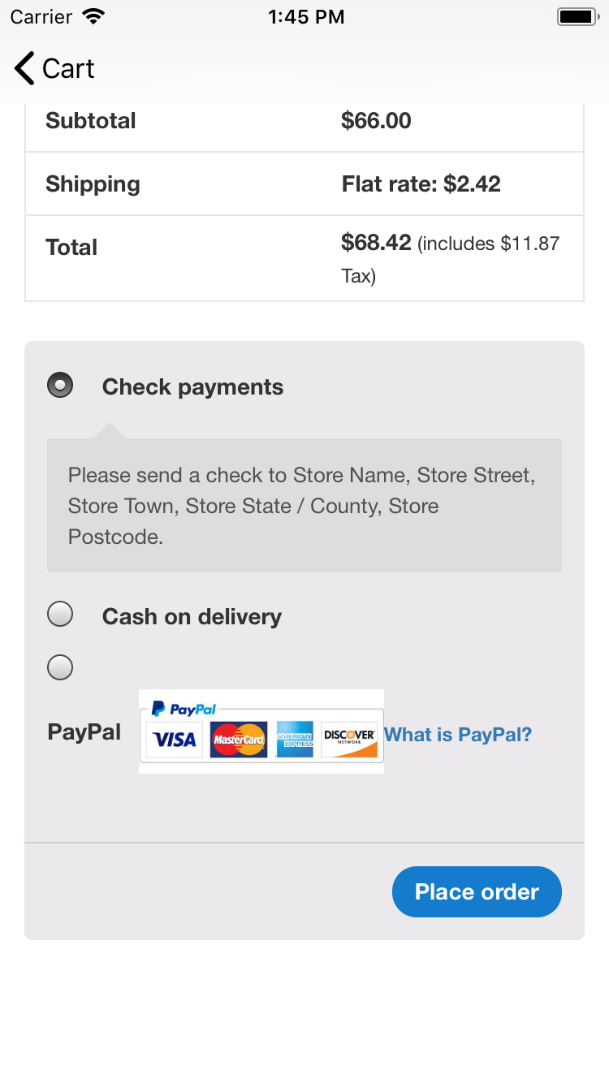This image is a detailed screenshot of a payment page on a mobile device. The top section of the screen, approximately one inch high, has a light bluish-gray background. Below that, a two-inch white section appears, followed by another light bluish-gray section extending to the bottom of the screen.

In the top left corner, the text "carrier" appears in black, and nearby, a fully active Wi-Fi icon is visible. The time "1:45 PM" is displayed in black text, followed by a full battery icon, also in black, on the right side.

Below the word "carrier" is a large greater-than symbol (">") pointing to the left. To the right of this symbol, "car" is written in black text. The white section beginning below this point contains a breakdown of costs: 
- "Subtotal" on the left, with "$66" on the right,
- "Shipping" below, with "Flat rate $"242" on the right,
- "Total" on the left, and "$68.42" on the right, which includes "$11.87" in total tax.

The light bluish-gray background resumes below this breakdown. Within this section, a small black circle with a white interior is positioned near text reading "Check payments." A tab pointing up towards "Check payments" displays black lettering that instructs, "Please send a check to store name, store street, store town, store state/counties, store postcode."

Further down, there are options for different payment methods:
- An outline of a circle labeled "Cash on Delivery" on the right of the first circle,
- An outline of another circle below that,
- "PayPal" on the left side of the lower circle, and within a rectangle are logos for PayPal, Visa, MasterCard, American Express, and Discovery.

Next to this, a blue text notes "What is PayPal?"

On the bottom right corner of the screen, a blue tab contains white text stating "Place order."